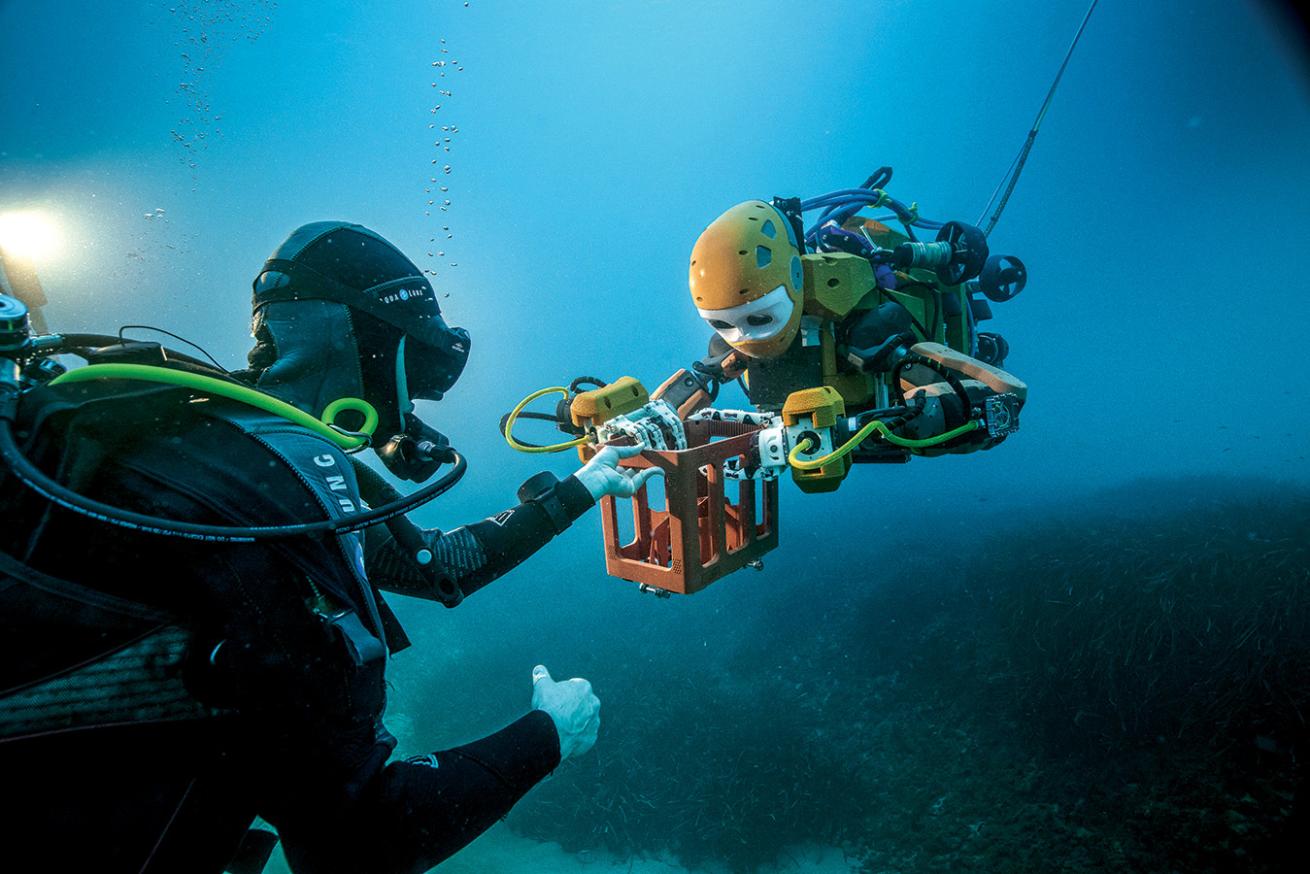In this detailed underwater photograph, two figures are depicted – a human diver on the left and a robot on the right. The human diver is clad in a black wetsuit, complete with an oxygen tank, goggles, and other essential scuba gear. They have their left hand extended, gripping a rectangular, brick-colored box. Opposite them, the robot, characterized by its entirely mechanical, metal body, is also grasping the same box. The robot's design includes a green body with a yellow helmet and a white mask over its eyes, resembling a human-face structure. The scene is set in the blue expanse of the ocean, with bubbles rising from the scuba diver and a dark, shadowy surface visible at the bottom right corner, indicating the seabed. The interaction between the human and the robot centers on the shared task of holding the brown box between them, highlighting a collaborative moment deep beneath the water’s surface.